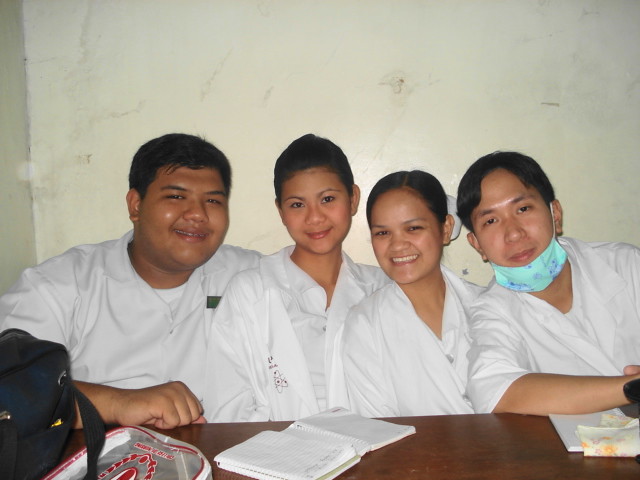In this photograph, a group of four young adults, who appear to be of Asian ethnicity, are seated around a dark brown wooden table. They are all smiling, exuding a sense of camaraderie. The backdrop features a dingy, yellowish wall with visible stains, adding a touch of grittiness to the scene. 

The man on the left has short black hair and a cheerful smile, with his left arm resting on the table. Next to him, two women with short black hair are seated. The woman closer to the left sports pink lipstick and a smile, while the woman to her right, who has a white scrunchie in her hair, also smiles broadly, revealing her teeth. Both women have brown eyes.

On the rightmost side sits another man with short black hair, parted in the middle, and a light blue face mask with dark blue spots pulled down to reveal his face. His hands rest on the table. All four individuals are wearing white—a mix of what might be lab coats or nurses' uniforms, suggesting a professional or academic setting.

The table holds various items, including a navy blue bag, a clear white and red bag, a black lunchbox, some notebooks, and food wrappers, hinting at a casual, possibly study-related gathering.